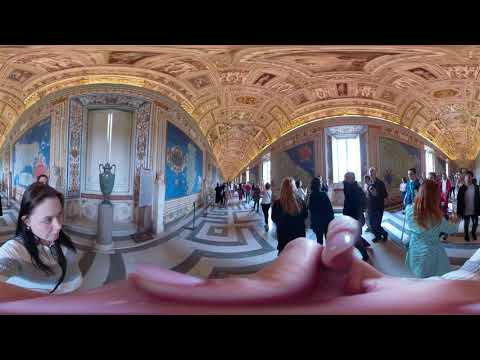This image provides a distorted fisheye view of an ornate and possibly historical building, most likely an art museum, cathedral, or palace, given the opulent architecture and artwork visible. The scene is bustling with a good number of pedestrians, many of whom are wearing jackets, indicative of cooler weather. The left side of the image features a woman with long brown hair wearing a white and gray striped shirt. Her hand is notably distorted, highlighting the use of a 360-camera that warps the surroundings, giving the entire image a surreal, curved appearance.

The building's detailed ceiling, which has a grand, cathedral-like design with gold and amber embellishments, arches impressively from the top. Several blue walls adorned with ornate designs and multiple framed portraits and paintings, some of which appear to be maps, enhance the indoor scenery. Natural daylight streams through visible windows, adding a touch of warmth to the scene. 

On the left side, a white marble pillar holds a distinct green vase with handles, adding to the grandeur. The floor stands out with its intricate, geometric pattern in green and white tiles, resembling a maze. This richly decorated interior, teeming with visitors, suggests a space of significant cultural or historical interest.